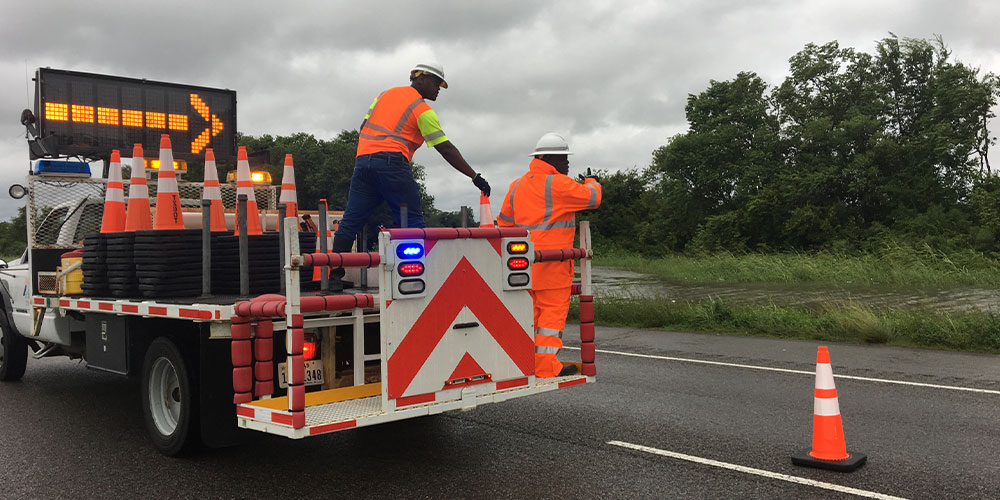This daytime photograph depicts a scene on a roadway involving two construction workers of brown skin tone and clad in safety gear. One worker, dressed in an orange full suit with reflective tape, stands on a lift attached to the back of a white utility truck, while the other worker, wearing a bright yellow T-shirt and orange vest, positions road cones on the ground. Both workers are equipped with hard hats. The utility truck, reminiscent of a modified pickup truck, features a digital sign with a yellow arrow directing traffic to the right, indicative of lane diversion typically seen during road construction or accidents. The truck's warning lights are activated, and the bed is loaded with numerous orange cones, one of which is already placed on the road to the right. The background reveals a high water level in what appears to be a river or runoff creek flanked by tall grasses, hinting at possible recent rainfall or flooding. The sky looks cloudy and windswept, suggesting the presence of stormy weather. Trees can be seen further in the distance, completing this detailed depiction of roadway safety activity amidst potentially adverse weather conditions.